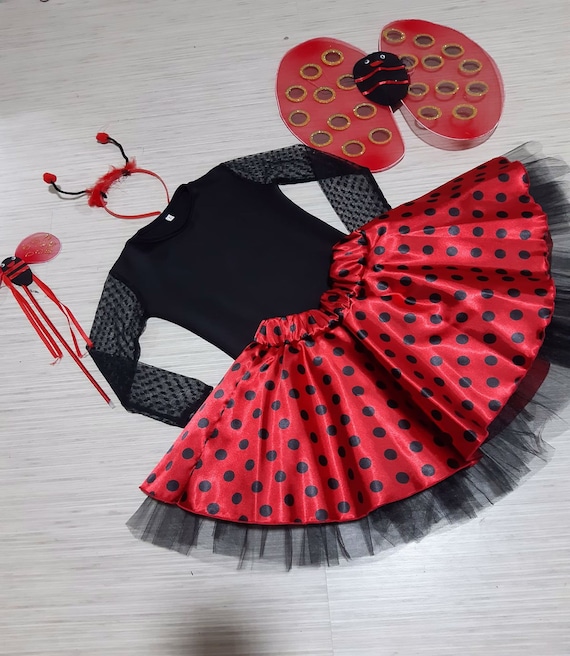The photograph captures a detailed portrait of a little girl's ladybug costume laid out on a light gray, possibly linoleum, floor. The ensemble includes a black long-sleeved top with semi-sheer gray sleeves adorned with little black dashes. Complementing the top is a vibrant red satin skirt, highlighted with black polka dots and edged with black lace. The costume also features dramatic accents: a pair of red ladybug wings situated in the upper right corner with gray polka dots outlined in gold foil and a central black oval with red stripes and googly white eyes. Above the top is a headband fitted with black antennae ending in red bulbs, mimicking a ladybug's look. Positioned to the left of the shirt, there's a whimsical wand with red and black ladybug details and flowing red ribbons. The entire outfit, likely intended for a Halloween costume or a dance recital, is arranged at an angle from the top left to the bottom right of the image.